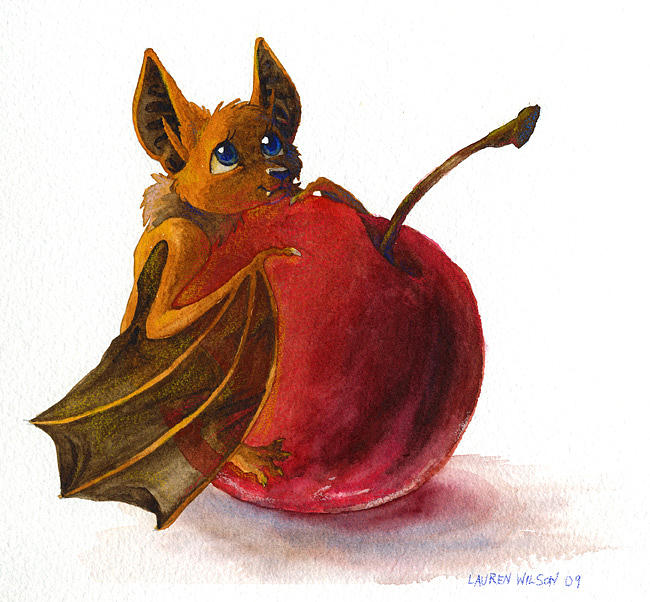The image showcases a detailed watercolor painting, set against a pristine white background. In the lower right-hand corner, the artist's signature, "Lauren Wilson, 09," is delicately inscribed in pencil, indicating the artwork's creation date in 2009. The focal point of the painting is a crimson-colored fruit, likely a cherry due to its long, brown stem that curves slightly upward and to the right, adorned with black and white shading that adds depth to its appearance. Clinging to the fruit on the left side, a cartoonish brown bat is depicted with striking blue eyes, a black nose, and a small white fang peeking from its mouth. The bat's ears are brown with black inner details, and its wings display dark, translucent webbing between light brown spines. Additional pink and purple shading enriches the surface beneath the fruit, enhancing the visual texture of the artwork.